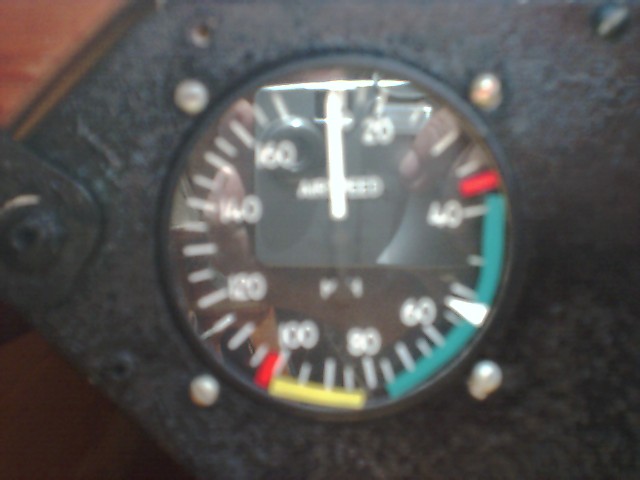A detailed rectangular photograph captures a round, centrally positioned gauge set into a sleek black frame. The gauge itself features a black facing adorned with numerous white lines marking the edges and extending inward. White numbers are evenly spaced at particular intervals around the gauge. A prominent white needle currently points to the top center, partially obscuring some blurred white text in the background. On the bottom right of the gauge, green lines are visible, while a yellow line is present at the bottom center. The entire gauge is securely mounted to a metal black plate with four shiny silver bolts. The reflective surface of the gauge's plastic or glass covering shows a faint reflection of the photographer. This black plate rests on a flat brown surface, providing a stark contrast to the sophisticated design of the gauge.